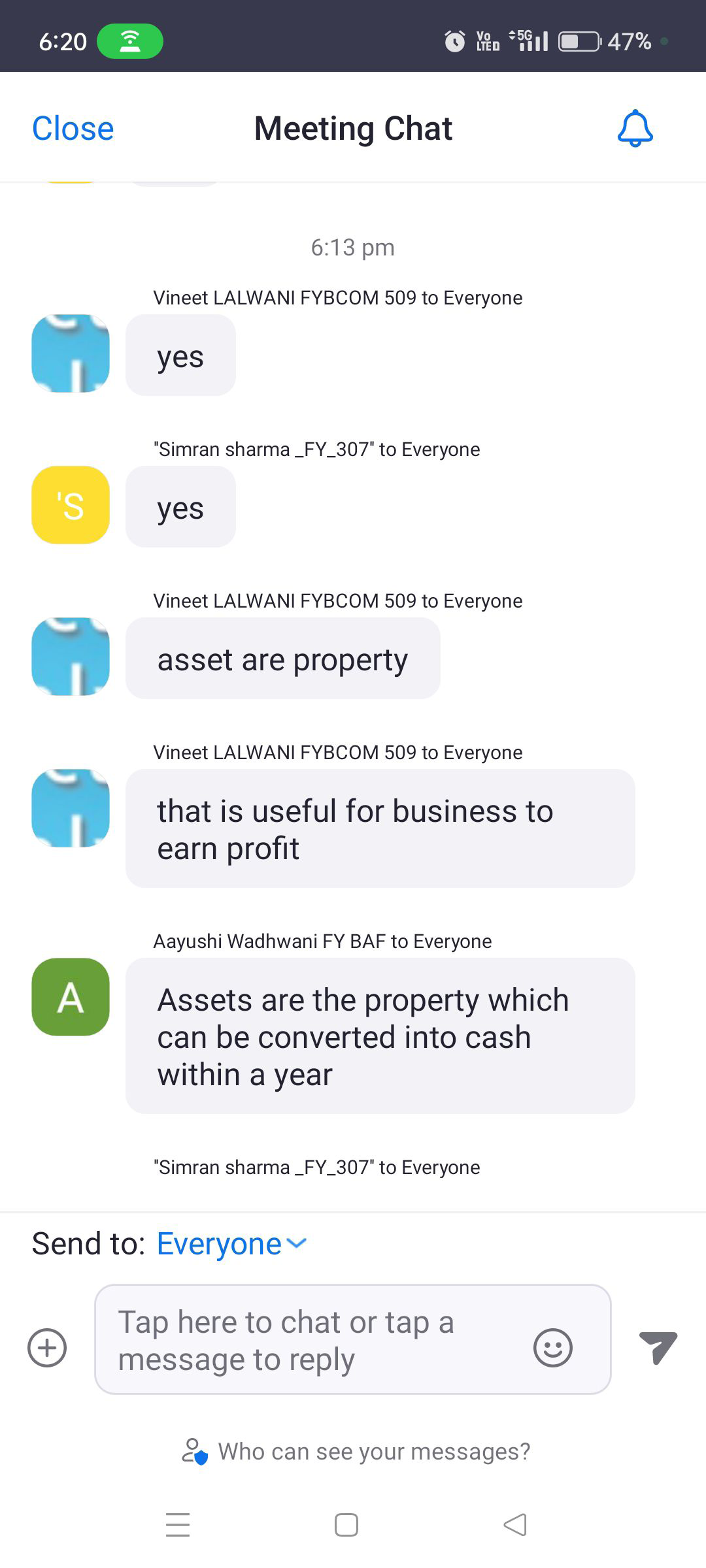The image is a screenshot from a meeting chat displayed on a mobile phone. The phone's taskbar at the top of the screen is black, featuring the current time (6:20), a green Wi-Fi icon, an alarm clock icon, a 5G status icon, and a battery indicator showing 47% battery life.

Beneath this black bar, the rest of the screen has a white background. In the top left corner of this section, there is a blue close button. Slightly to the right, the words "Meeting Chat" are displayed in black text, accompanied by a blue bell icon to the right.

The chat conversation begins with a message timestamped at 6:13 PM from Vineet Lalwani FYBCOM 509, who addresses everyone in the chat. Vineet's message reads, "Yes." Each participant in the conversation is represented by a colored icon: blue for Vineet, yellow with a white "S" for Simran, and green with an "A" for Ayushi.

Following Vineet's initial message, Simran Sharma responds to everyone with a simple "Yes." Vineet then sends two more messages, the first stating "Asset or property" and the second elaborating, "That is useful for business to earn profit."

Ayushi Wadwani FYBAF subsequently contributes to the conversation by stating, "Assets are the property which can be converted into cash within a year."

At the bottom of the screen, there is a text box labeled "Send to" with the word "everyone" in blue and a small down arrow next to it. Below this, there is a field for entering a new message, indicating where the user can type their response.